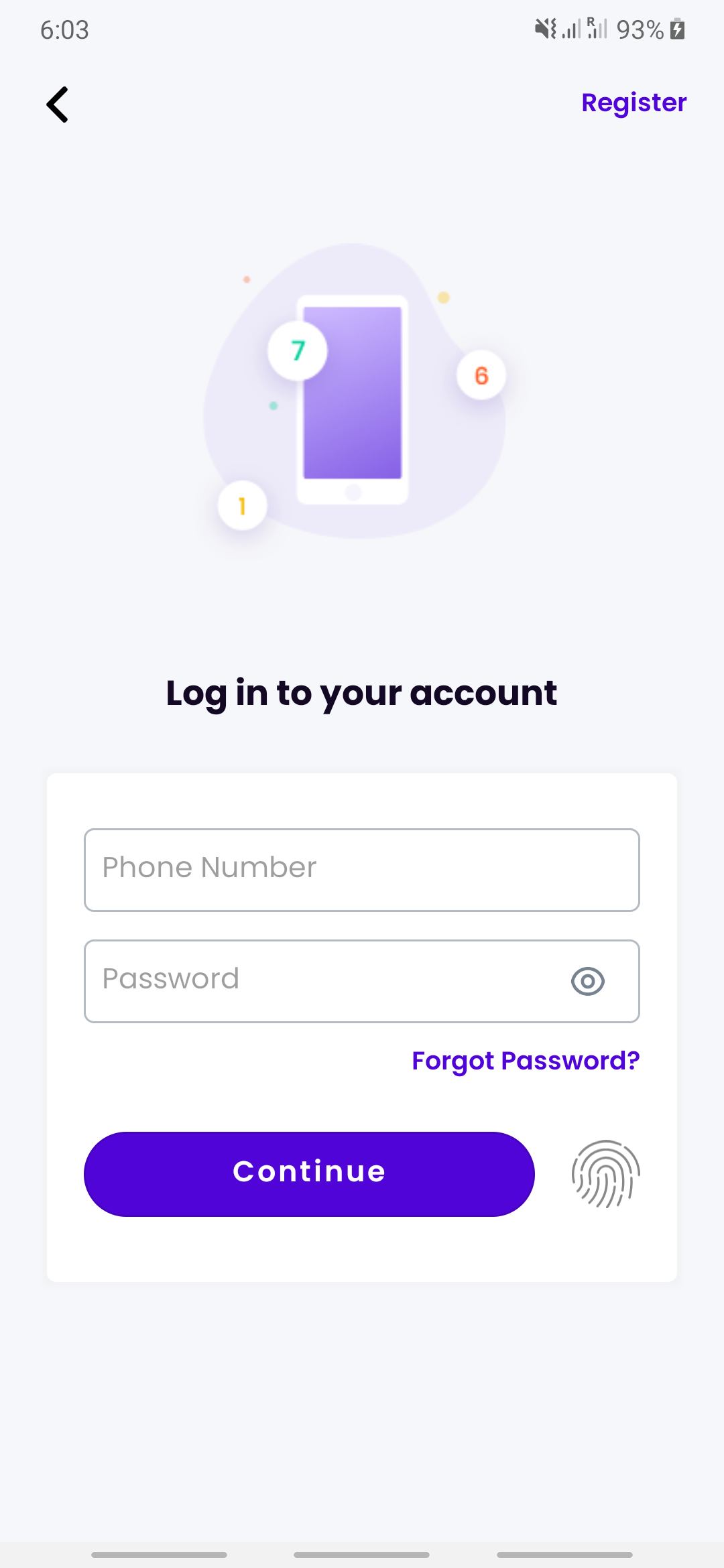This is a detailed screenshot of a login page displaying a user interface with various features and elements. The background screen is primarily gray. In the top left corner, a black back arrow is visible, allowing users to navigate to the previous page. Adjacent to it on the right, there is a purple "Register" button. Below this, a purple screen features a smartphone icon illustrating the UI. Within this icon, several numeric indicators in white circles are present; a yellow circle with the number 1, a green circle with the number 7, and a red circle with the number 6.

Directly below the icon, the text "Log into your account" is prominently displayed in black. Beneath this, there is a white input box containing two fields. The top field is labeled "Phone number", and the bottom field is labeled "Password". An eye icon button is located to the right of the password field to toggle visibility. Positioned underneath these fields, to the right, the text "Forgot password" is displayed in purple, providing a recovery option.

Further down, on the left side, a prominent purple pill-shaped button labeled "Continue" is available for users to proceed with logging in. To the right of this button, there is a fingerprint icon implying biometric login capability. The remainder of the background maintains a consistent gray color.